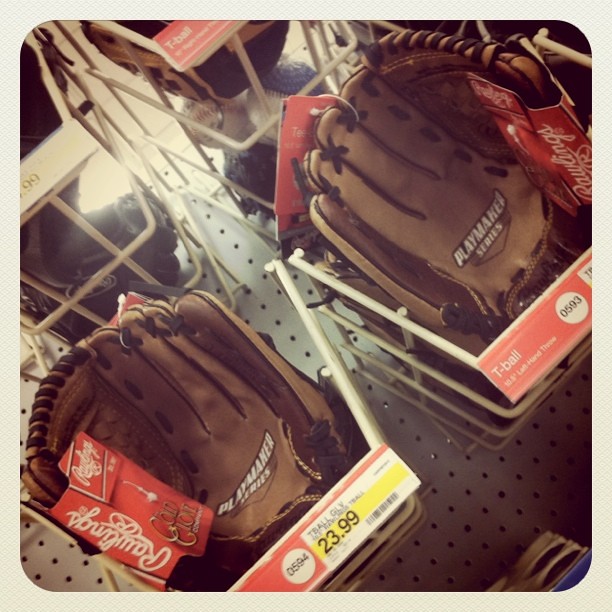The image depicts a detailed and organized display of Rawlings baseball gloves at a department store. Each dark brown leather glove sits in its own white metal basket, hooked onto a pegboard with a brownish hue. The pegboard's perforations suggest it's a versatile hook slot setup, commonly used in stores. The gloves feature a bright red and white Rawlings tag looped near the finger area, reinforcing their branding. A yellow-highlighted price tag reading $23.99 is attached to the metal frame of each basket, indicating each glove's price. The metal frames and the pegboard itself are positioned so that they can be accessed from either side of the aisle, making the display easily approachable for shoppers.